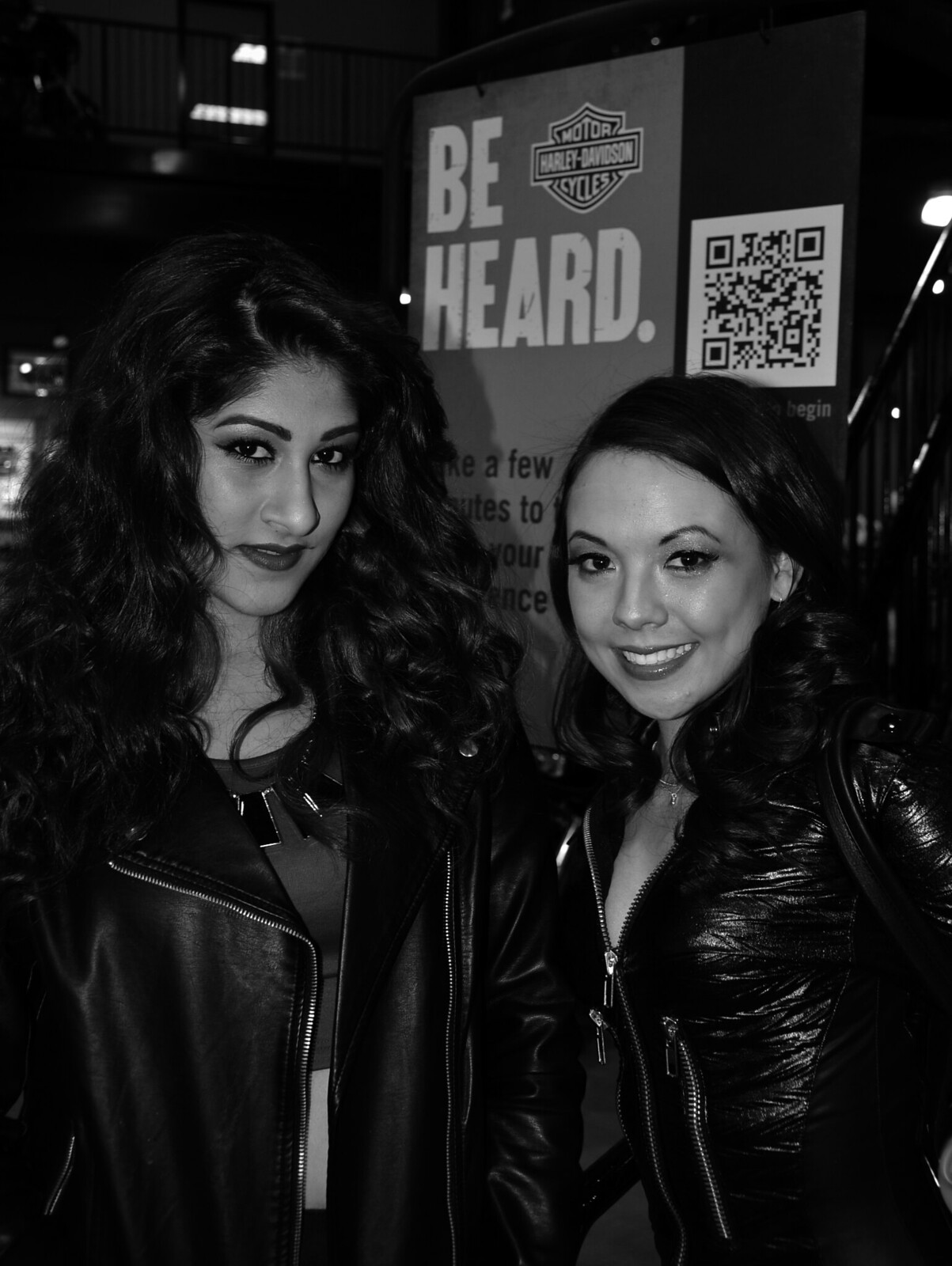In this black-and-white photograph, two young women in their 20s or 30s, both wearing dark leather jackets and medium-colored shirts, pose side by side with their shoulder-length, curly hair either dark or appearing darker due to the filter. Both are heavily made up, with noticeable lipstick and eye makeup, and each wears a necklace. One of the women is about eight inches taller than the other. They stand in the center of the image, looking directly at the camera — one with a smile, the other with a neutral expression. Behind them, a poster bearing the Harley-Davidson Motor Cycles logo and the slogan "Be Heard" is visible, along with a QR code. The setting appears to be indoors, possibly at an expo or convention, hinted by the presence of a balcony and stairwell in the background. The overall scene is meticulously composed, emphasizing the women and the iconic brand association, presented in varying shades of gray.